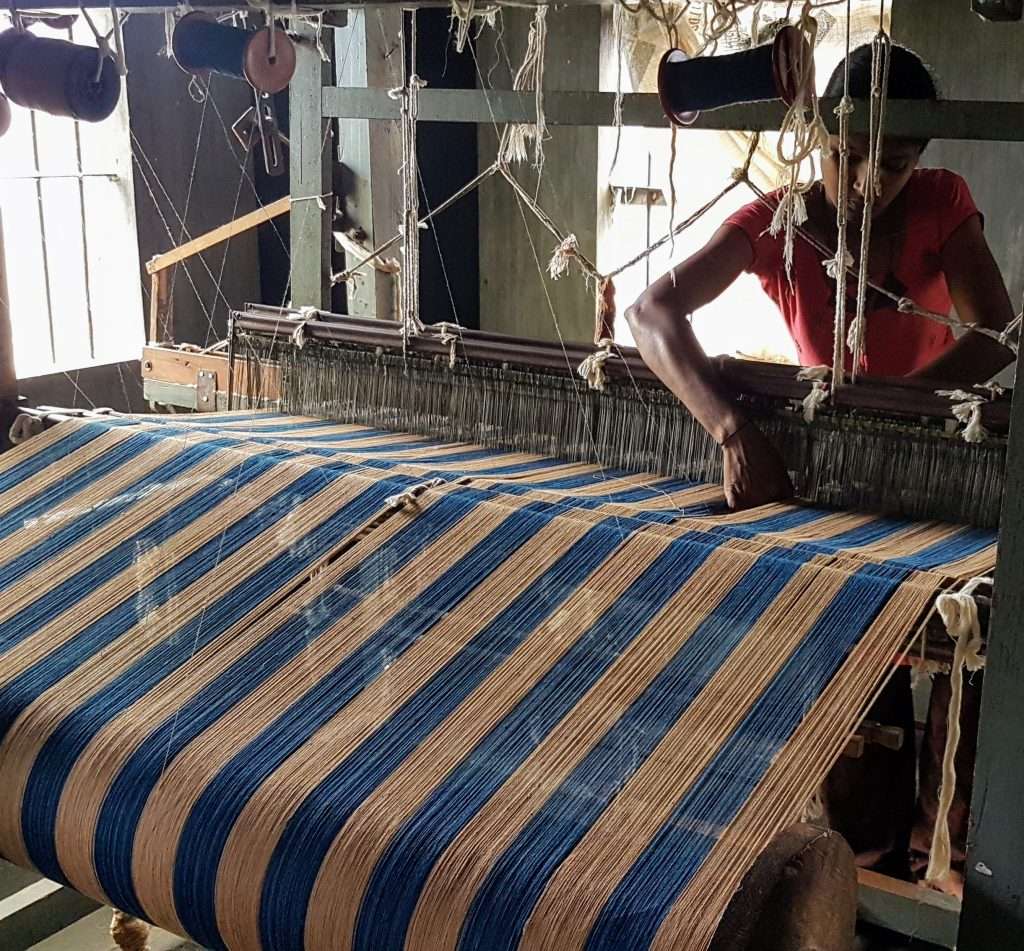The image depicts a woman operating a mechanical weaving device to create a textile with alternating blue and brown stripes, each comprising several threads or strands of yarn. She stands behind the machine, reaching over it to adjust the yarn material, ensuring it aligns correctly. The woman, dressed in a red T-shirt and possessing dark skin, is positioned in a well-lit room with sunlight streaming in from a barred window and a door on the upper left side. Above the machine, numerous strings and spools of yarn are visible, contributing to the intricate process.